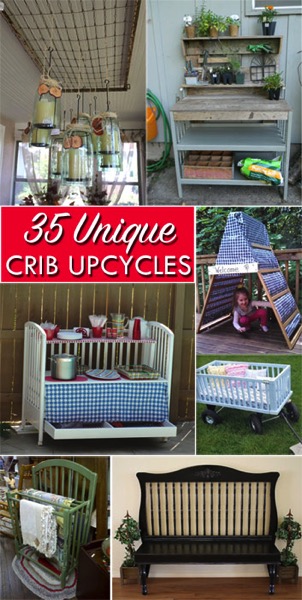The image features a collage of various photographs, each depicting innovative ways to repurpose old cribs. Central to the image is a bold caption with a red background and white lettering that reads "35 Unique Crib Upcycles." Notable transformations include a wooden bench crafted by converting parts of the crib, a wagon with wheels added to the base, and a shelf assembled from half of a disassembled crib. Other inventive uses shown are a black bench that uses the crib's side as a backrest, a towel hanger utilizing the crib's rungs, and a playful tent for children. Each small picture highlights a unique and creative way to give new life to an unused crib.